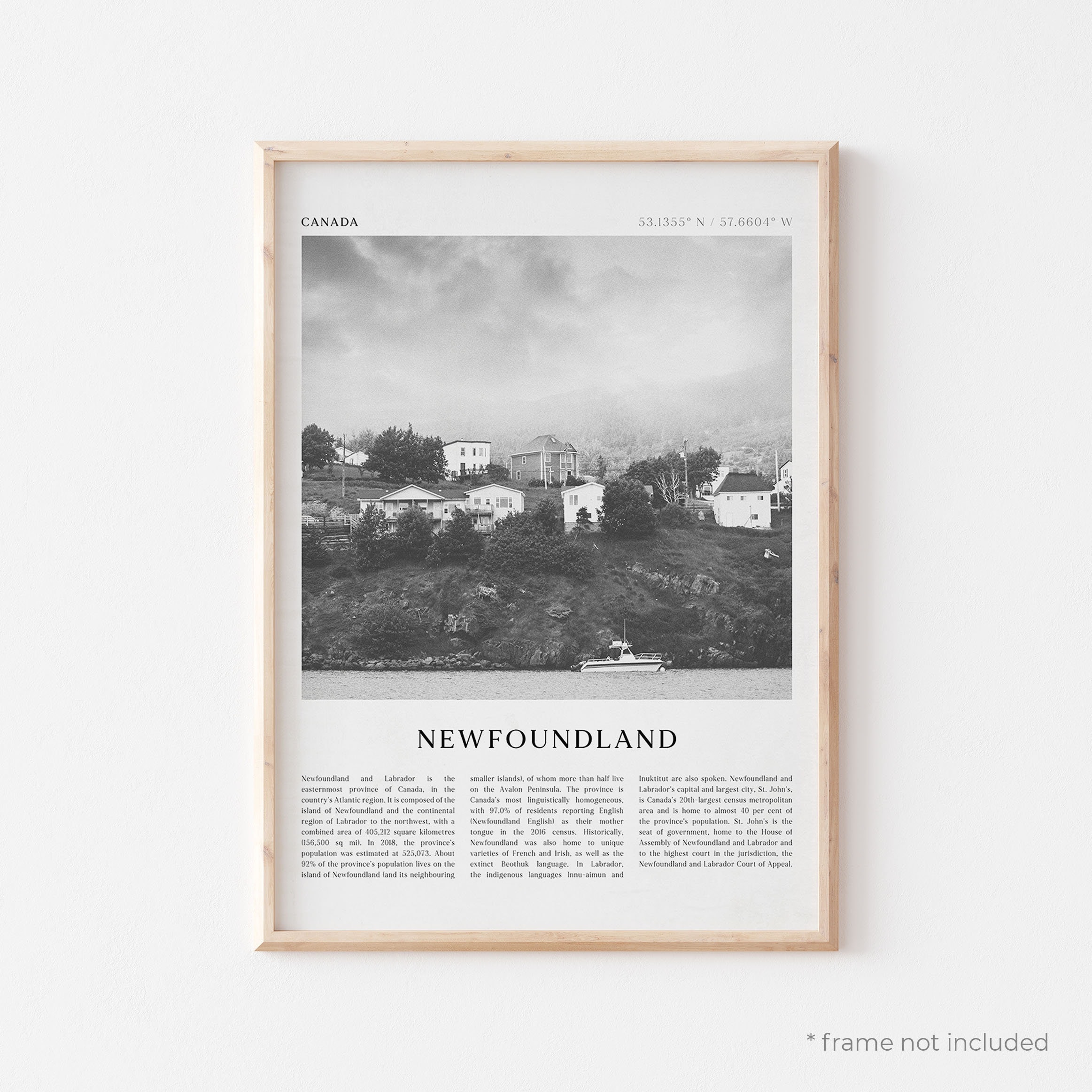A framed black and white poster of Newfoundland, displayed against a white wall, captures the essence of this historic location. The light brown wooden frame elegantly encases the image. At the top of the poster, the word "CANADA" is prominently displayed on the left side, while the geographic coordinates, 53.1355° N and 57.6604° W, are subtly noted on the right. The photograph itself portrays an overcast sky with ominous clouds hovering over a craggy hillside dotted with several small homes and greenery. The foreground reveals the calm waters of the Atlantic Ocean with a solitary boat. Below the image, the title "NEWFOUNDLAND" is boldly printed, followed by three columns of diminutive, almost unreadable text that likely describes the area's history and features. The bottom right corner of the image outside the frame includes a small asterisk and the note "*FRAME NOT INCLUDED," suggesting it's a purchasable item. The overall composition evokes a sense of timeless tranquility and historical depth.